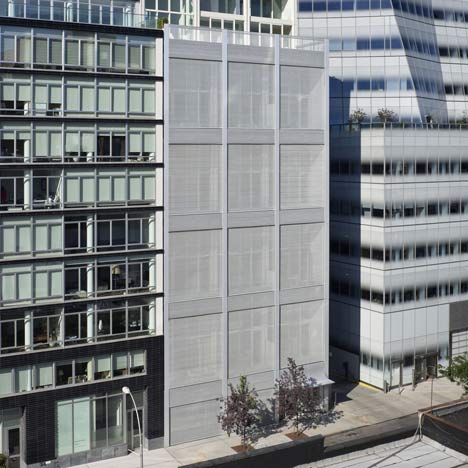This image captures three tall buildings in a city, viewed from a building across the street, emphasizing their height and urban environment. The buildings feature large, glass windows, and their modernity is highlighted by distinct architectural details and varying window treatments. The structure on the left has numerous glass windows with black frames, some adorned with white curtains. The center building bears a dark gray mesh-like covering, giving it a sophisticated appearance, while the one on the right stands out with its white facade accented by black and blue windows. There are two trees with maroon and green leaves in front of these buildings, casting hard shadows under the midday sun. Below, a gray sidewalk and a ground area with netting, possibly a sports court, stretch across the front, further enhancing the urban atmosphere. The overall color palette includes shades of gray, white, and hints of blue, with the vibrant foliage adding a splash of color to the scene. The image, taken from a considerable distance, offers a panoramic view of the cityscape, capturing the essence of urban living and the juxtaposition of different architectural styles.